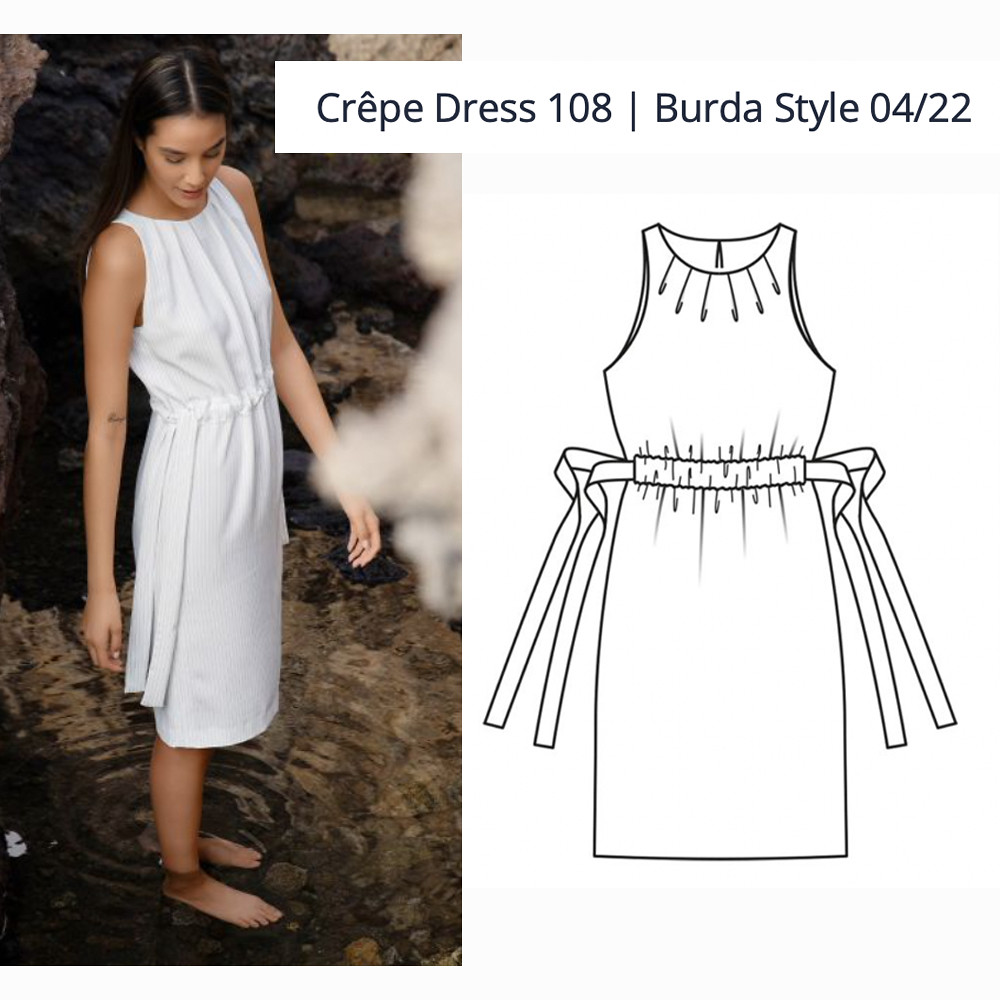The image appears to be an advertisement for a white crepe dress, designated as Crepe Dress 108, and Burda Style 04-22. The headline at the top reads "Crepe Dress 108," while to the right, it says "Burda Style 04/22." The image features a black-and-white diagram of the dress design on the right-hand side, showcasing the dress's pattern in a simple, 3D drawing. On the left-hand side, a slim, dark-haired woman models the dress, giving a practical view of how it looks when worn. Barefoot and standing in a small puddle or stream of water, she exudes a summery vibe, highlighting the casual and comfortable nature of the dress. The dress includes a belt strap at the midsection, adding to its simplicity and elegance. The overall composition of the advertisement effectively combines the detailed pattern diagram with a real-life depiction, making the dress accessible and appealing.